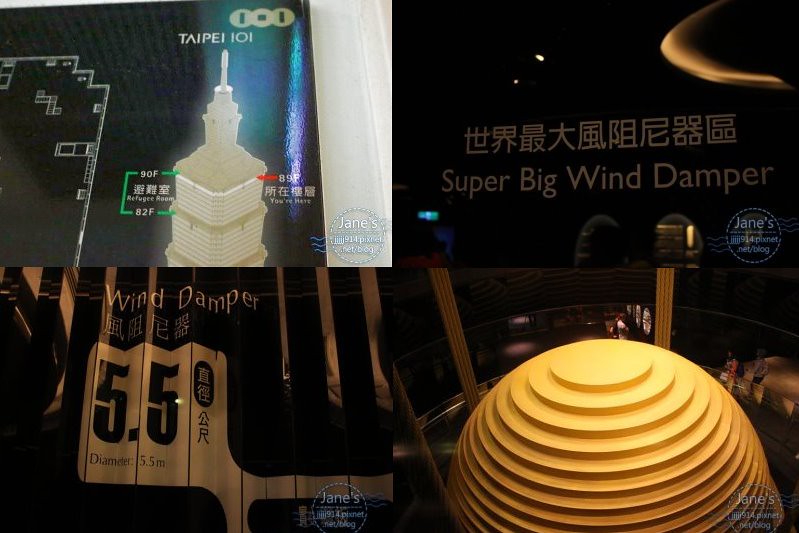This composition appears to be a detailed informational poster, potentially an architectural diagram, subdivided into four quadrants. The upper left quadrant features an architectural rendering of a tall skyscraper, likely the Taipei 101, with its structural design annotated in green and red arrows. Accompanied by Chinese characters, the text on a black background with light brown font reads "super big wind damper.” Below, the lower left quadrant depicts a fan-like text arrangement that includes both Chinese characters and the English term "wind damper," along with the numeric value 5.5. The lower right quadrant showcases a geodome or hemisphere formed by concentric circles illuminated in golden yellow light. Each quadrant bears a watermark in the lower right corner reading 'Jane something,' implying authorship or copyright. The overall poster appears informative, possibly explaining the functionalities of wind dampers within the skyscraper, incorporating multilingual annotations and architectural visuals.